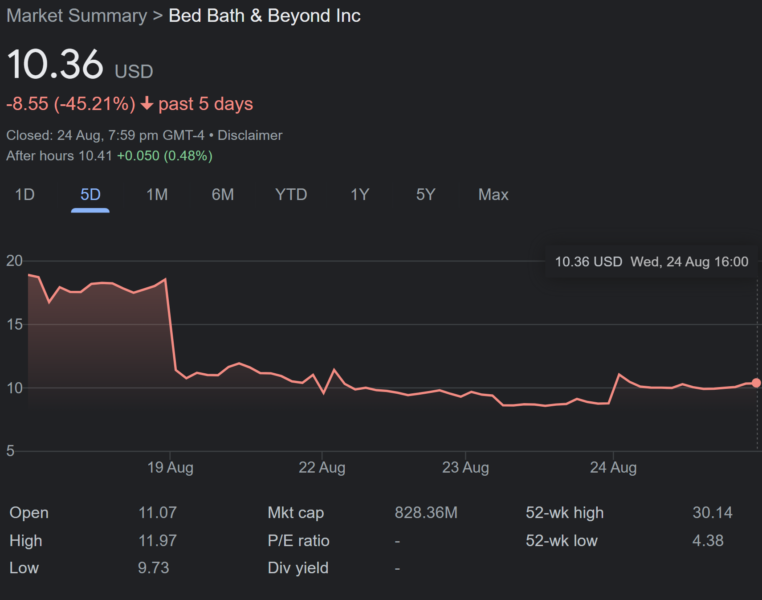In this detailed stock market screenshot, the black background prominently features a market summary at the top in light white font, indicating "Bed Bath & Beyond Inc." The stock price, $10.36 USD, is displayed just below in a lighter white shade for "USD." A striking orange display shows a decline with "-8.55" and "-45.21%" accompanied by a downward-pointing orange arrow indicating a significant drop over the past five days. Below this, in a grayish font, it is noted that the market closed on "24 August, 7:59 PM, GMT-4," followed by a small dot and the word "disclaimer."

Further down, the "after hours" price is marked at $10.41, with a green indication of a slight increase "+0.050" (0.48%). The timeframe options for the stock's performance are listed in sequence: "one day," "five day" with a blue underline, "one month," "six months," "YTD," "one year," "five year max," with the latter options in gray.

The chart beneath displays price levels marked as 20, 15, 10, and 5, with an orange trendline beginning around 20 and currently settling just above the 10 mark. On the right side, additional stock details are displayed, beginning with "$10.36 USD" on Wednesday, August 24th, at 16:00. Below this, key dates "August 19th, August 22nd, 23rd August, 24th August" are listed.

Further information includes the opening price of "11.07," market capitalization "828.36 million," and the 52-week high "30.14." The following lines provide specifics such as the day's high "11.97," P/E ratio, which is marked with just a tick, the 52-week low at "4.38," and the day’s low at "9.73." The dividend yield is simply indicated with a dash.